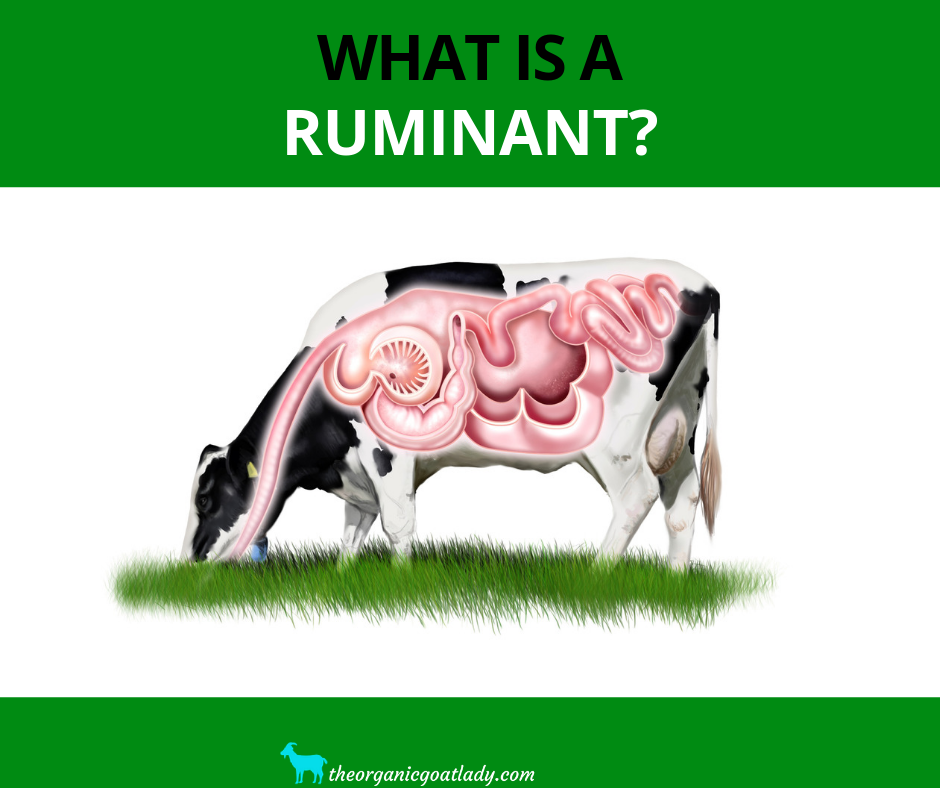The image features a detailed diagram of a ruminant's digestive system. At the top, a vibrant green horizontal rectangle contains the title "What is a ruminant?" with "What is a" in black text and "ruminant?" in white. Below, the main section, set against a solid white background, showcases a black-and-white dairy cow in a left side view, its head lowered to graze on a bright green patch of grass. Notably, a pink outline details the cow's digestive tract, extending from its mouth through its body. The cow's head is mostly black with a white top, transitioning to a body that alternates between black and white patches. At the bottom of the image, another horizontal green rectangle displays the URL "theorganicgoatlady.com" in white italicized text, accompanied by a small turquoise blue goat icon to the left.